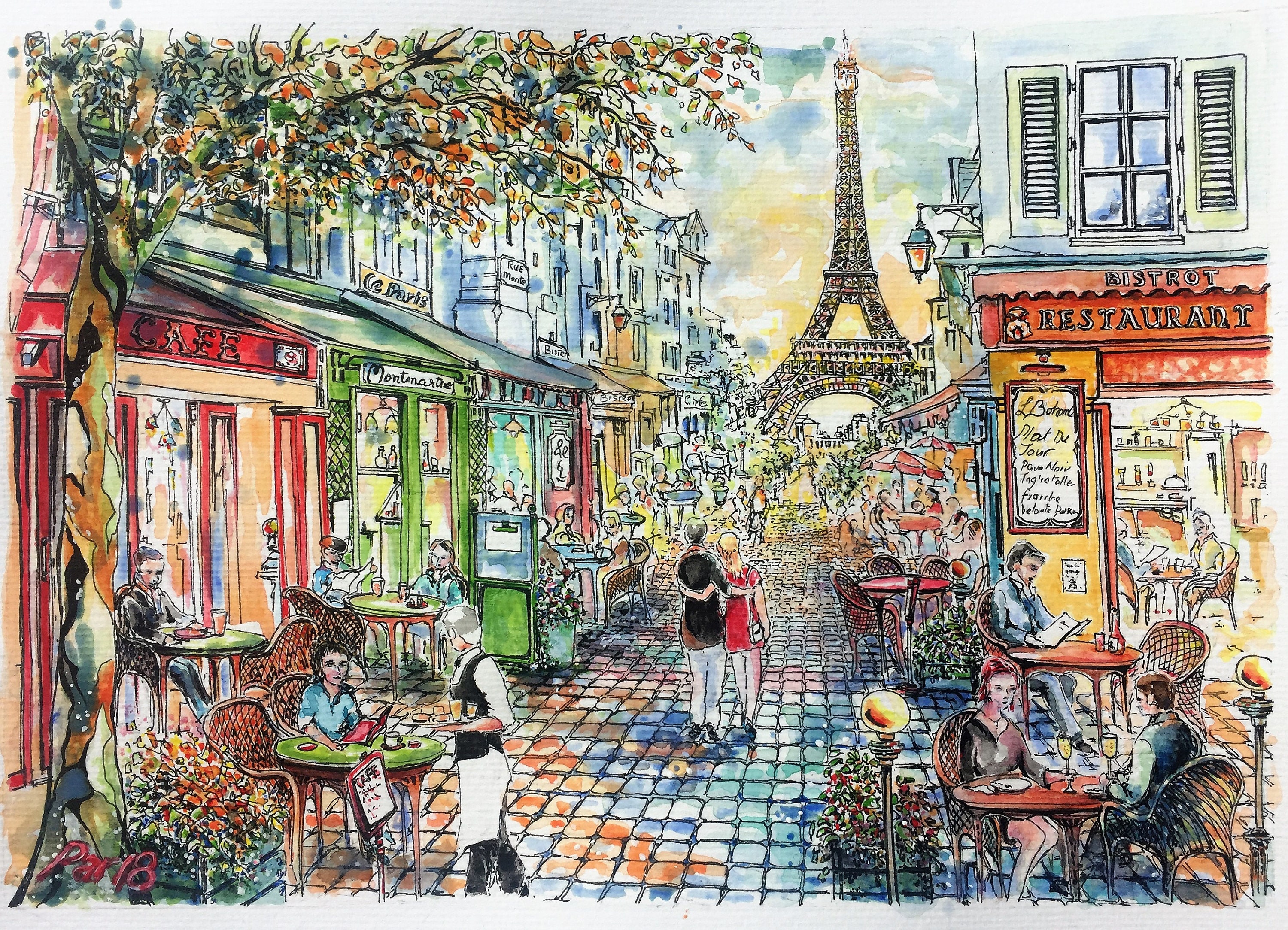This richly detailed illustration captures the lively essence of a Parisian street, bustling with activity and charm. The scene is set on a cobblestone street lined with colorful buildings, rendered in pen outlines with watercolor washes. The street leads towards the iconic Eiffel Tower, which stands prominently in the background, confirming the location as Paris. 

To the left, a little red cafe stands out among buildings of various hues—browns, greens, and others—where tables with street umbrellas provide shade for patrons enjoying the pleasant weather. There are people seated outdoors: two women having coffee and reading the paper, a single woman dining alone, and another being served a drink by a waiter.

At the center of the scene, a couple strolls arm in arm down the cobblestone street. The woman, wearing a red shirt and white pants, and the man, in a black jacket with a scarf and white pants, add a romantic touch to the image.

On the right-hand side, a bistro with an open door reveals both indoor and outdoor seating. Patrons include a man reading at a cafe, another couple savoring a glass of wine, and various others engaged in lively conversation or simply enjoying their meals. A menu lit by a small lamp adds to the quaint and inviting atmosphere.

Towering trees and a beautifully delineated sky enhance the sense of openness and delight, making it a picturesque Parisian street scene brimming with activity, color, and the timeless allure of the City of Lights.